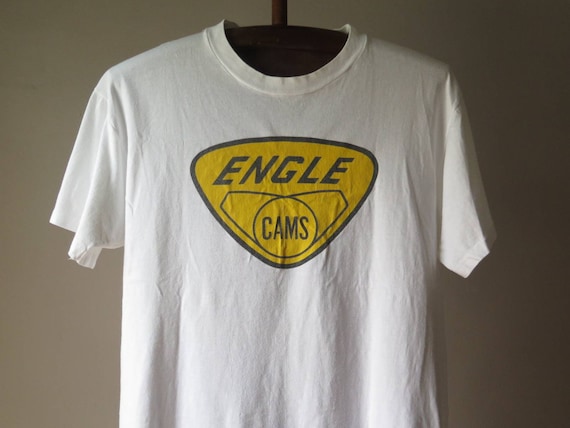This color photograph depicts a short-sleeved, crew neck white t-shirt hanging from a wooden, black clothes hanger against a brownish-gray solid background. The cotton t-shirt is notably wrinkled. Prominently displayed on the middle chest area of the t-shirt is a distinct logo. This logo is a yellow triangle with rounded corners, resembling an upside-down gumdrop or Hershey Kiss, and is outlined in black. Inside the triangle, "ENGLE" is written in large black letters, and below it, "CAMS" is inscribed in smaller black text, surrounded by two geometrical outline shapes.